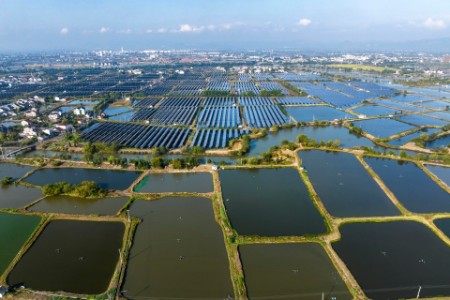This aerial photograph showcases an expansive landscape of rectangular plots inundated with water, bordered by strips of dry land. Prominent in the image are large arrays resembling solar panels that slightly reflect sunlight, positioned in rows across several plots. In the distance, the image captures small housing structures and a faint outline of a town or village, framed by suggestive silhouettes of mountains and clouds. The seemingly man-made ponds dominate the forefront, hinting at purposes ranging from water purification to rice farming or fisheries. The overall scene gives an impression of a meticulously organized land use system, viewed from a significant height, likely from an aircraft.